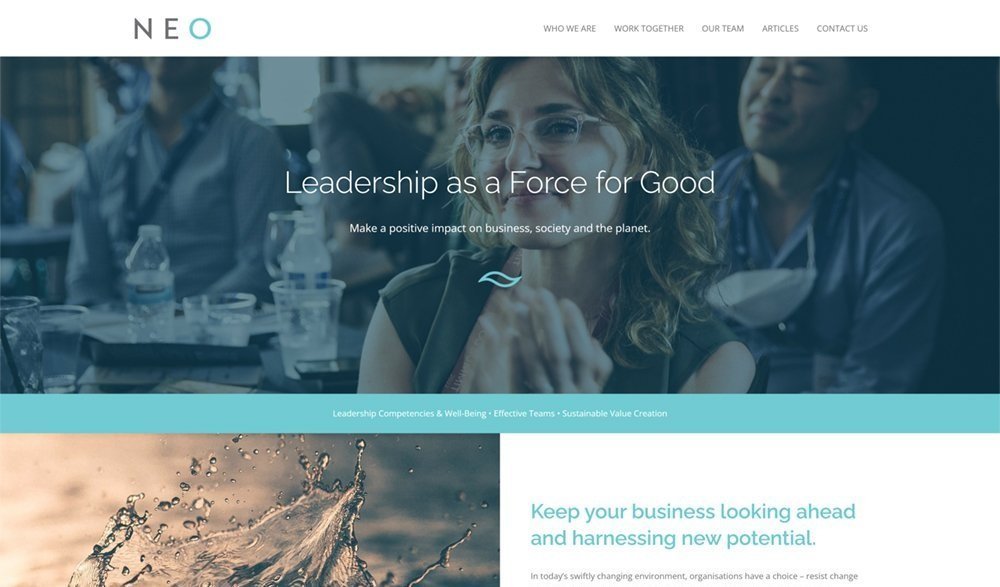The image is titled "Neo" with "N" and "E" in black and the "O" in teal. On the right side, text reads: "Who We Are, Work Together, Our Team, Articles, Contact Us." The background features a box filled with water bottles and disposable glasses. Men with lanyards and masks are present, with a woman in the foreground. The caption atop the image states, "Leadership as a Force for Good: Make a Positive Impact on Business, Society, and the Planet." Below, a floating teal piece of paper appears. A teal box beneath contains text on leadership, companies, well-being, effective teams, sustainability, and green initiatives. Underneath the box, there's a striking image of water splashing, capturing droplets and waves in midair. Adjacent to this, teal text reads, "Keep Your Business Looking Ahead and Harnessing New Potential. In today's swiftly changing environments, organizations have a chance to reset and resist change."